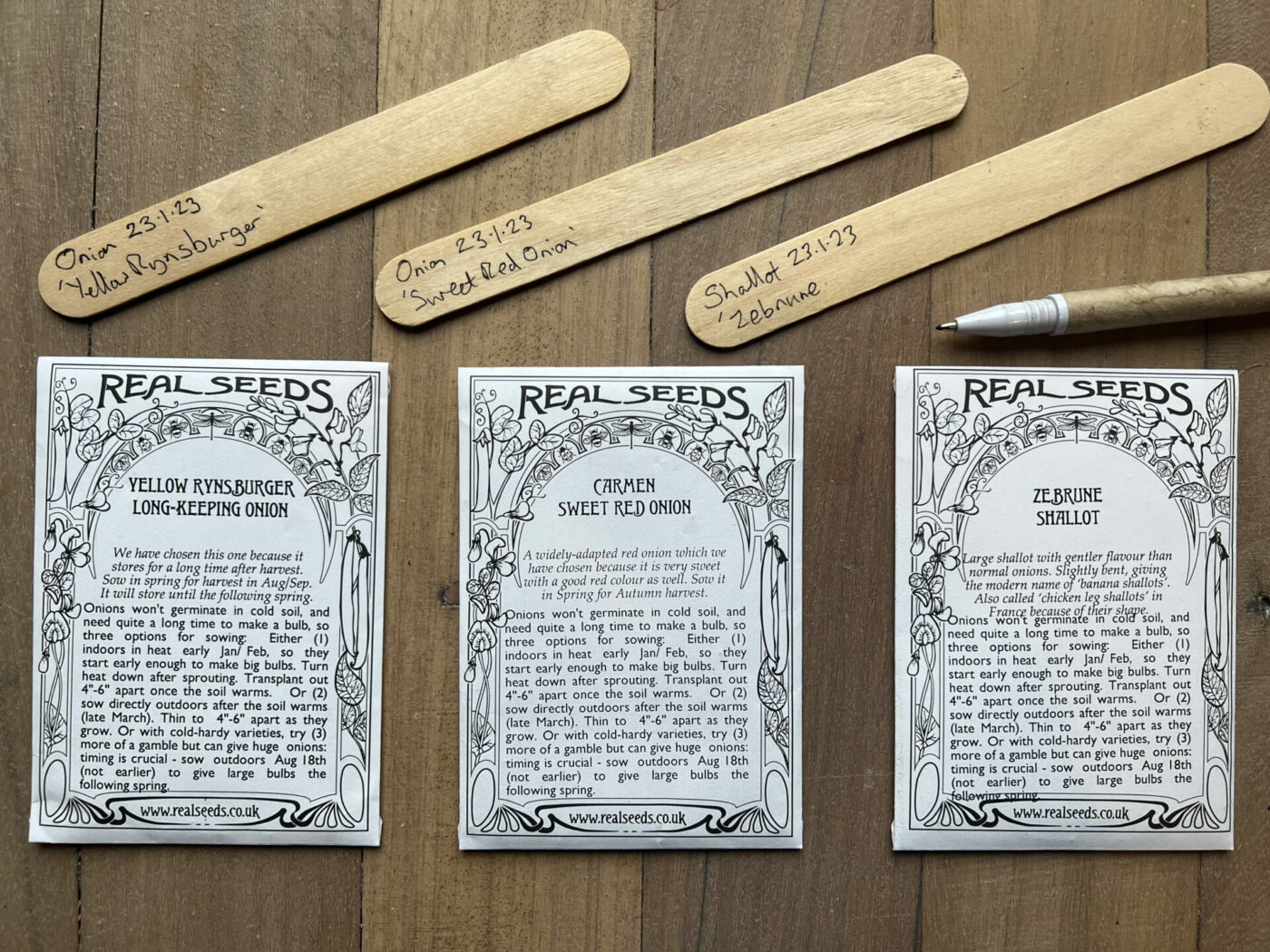The image features three antique-style black-and-white seed packets for different types of onions and shallots, neatly arranged on a wooden desk with vertical wooden panels. Each seed packet, adorned with floral and vine designs, prominently displays "Real Seeds" in black text. The packets are: "Yellow Rinsburger Long Keeping Onion," "Carmen Sweet Red Onion," and "Zebrune Shallot." At the top of each packet, a wooden tongue depressor, written by hand, identifies the type of seed and the date "23-1-23." Accompanying the seed packets is a pen with a white tip and wooden handle, used for labeling. These labeled sticks are typically used in gardens to keep track of planted seeds.